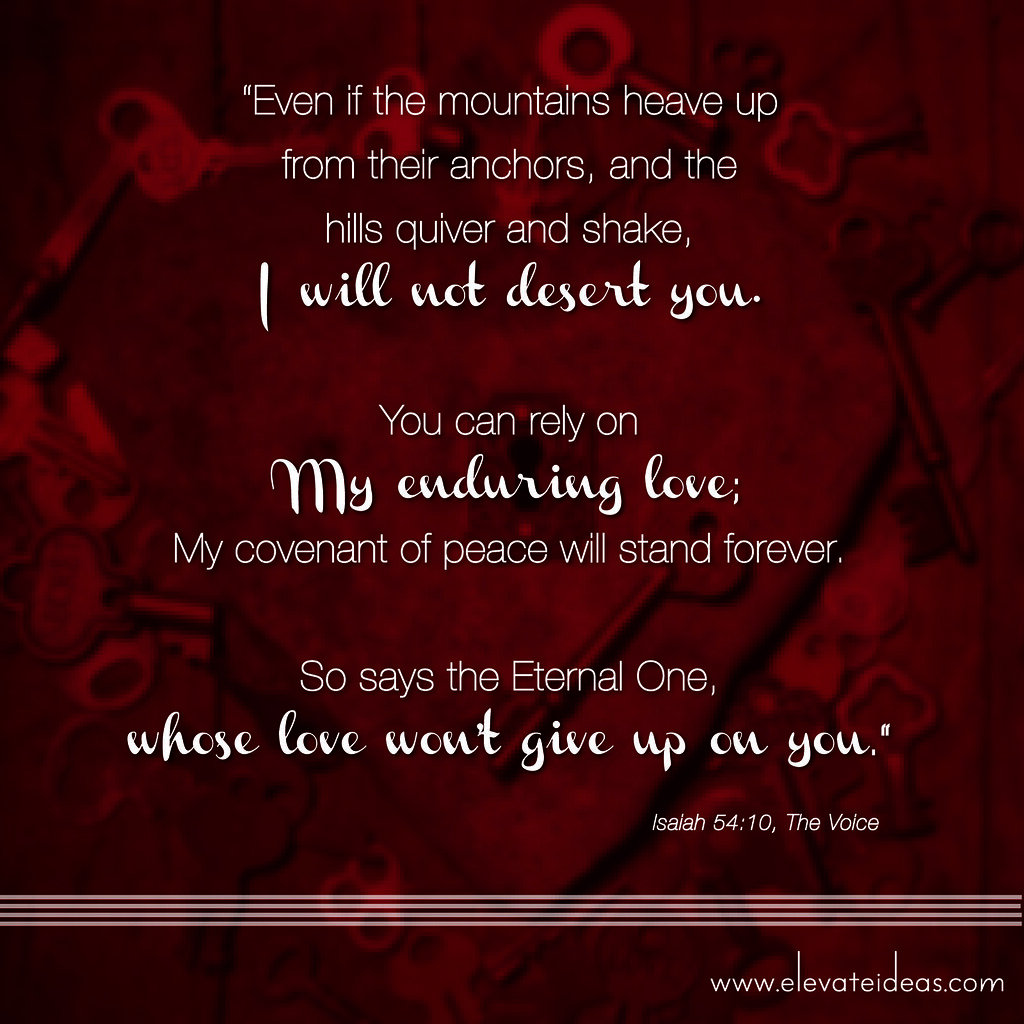The image features an inspirational quote set against a dark red background adorned with a faint heart shape and scattered keys. The quote reads, “Even if the mountains heave up from their anchors and the hills quiver and shake, I will not desert you. You can rely on my enduring love; my covenant of peace will stand forever. So says the Eternal One, whose love won't give up on you," attributed to Isaiah 54:10, The Voice. Key phrases within the quote—“I will not desert you,” “my enduring love,” and “whose love won't give up on you”—are highlighted in cursive, with a bolder, darker appearance. Below the quote, four horizontal white lines stretch across the image's width, and at the very bottom right corner, the text www.elevateideas.com is displayed.